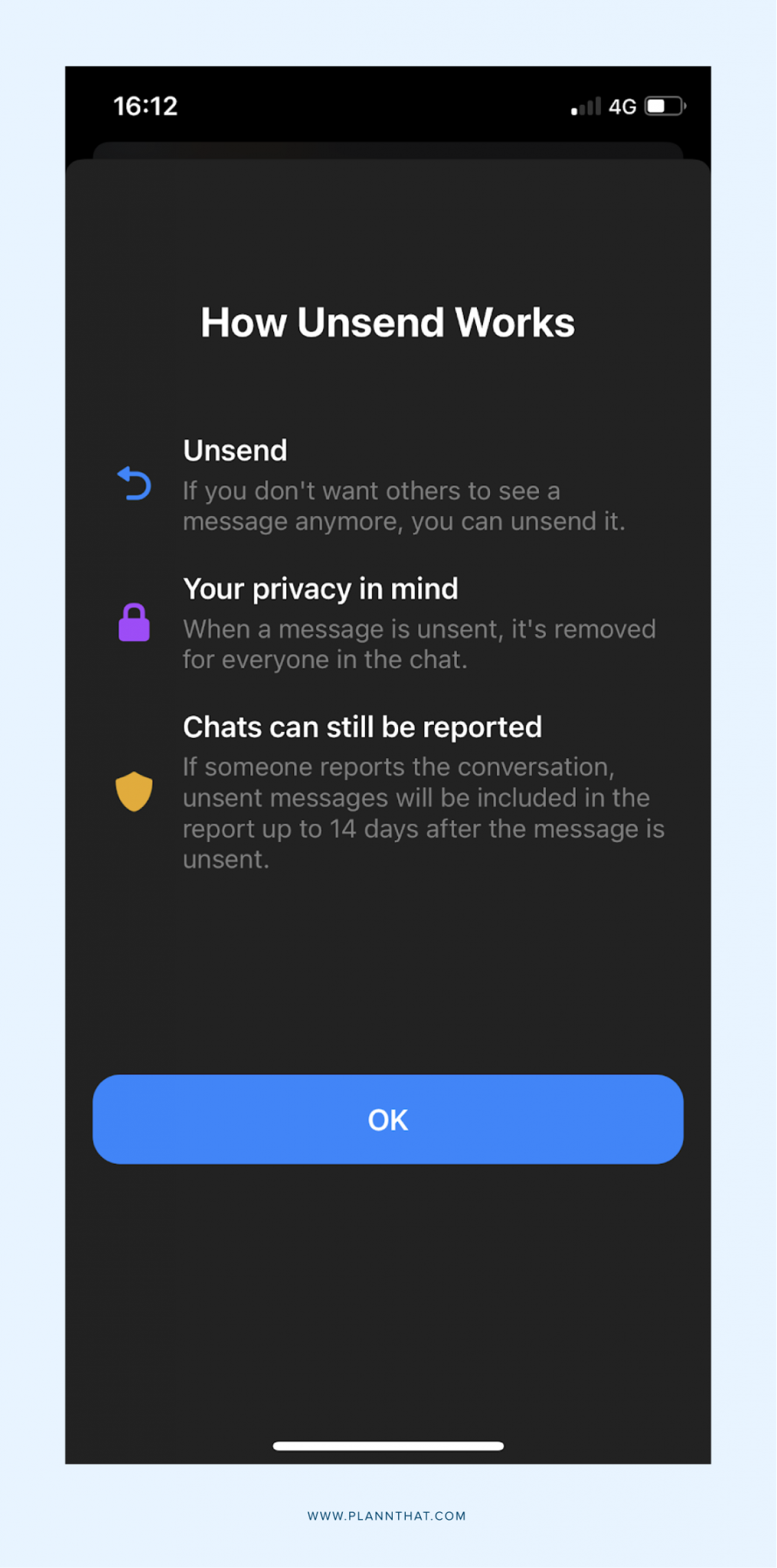The image displays a cell phone screen featuring a website with a light powder blue border. The URL at the bottom reads "www.plannthat.com" clearly spelled out. The website's background is black, and near the top, the white text displays the time as "16:12," along with indicators for a 4G network, battery level, and cell signal strength on the right side.

In the central part of the display, there is a bold white heading that reads "How Unsend Works." Beneath this, the word "unsend" appears next to a curved blue arrow pointing to the left. The text elaborates, explaining that users can unsend messages they no longer want others to see. Adjacent to a purple padlock icon, the message emphasizes the emphasis on privacy with the statement, "Your privacy in mind. When a message is unsent, it’s removed for everyone in the chat."

A gold shield icon follows, accompanied by an explanation in white text stating, "Chats can be reported. If someone reports the conversation, unsent messages will be included in the report for up to 14 days after the message is unsent."

At the bottom of the screen, there is a prominent blue button with the word "OK" in white print.